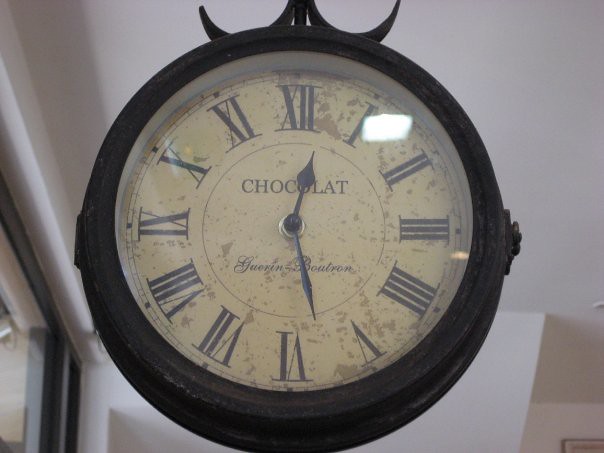The photograph features a close-up, slight upward angle view of a round clock suspended from the ceiling, though the exact mounting mechanism is out of frame. The clock's outer casing is a dark, almost iron, metallic color. The face of the clock has an aged appearance, with an off-white background speckled with gray and brown, resembling weathered parchment. The clock face prominently features Roman numerals in a light black or gray color, indicating the numbers 1 through 12. The time displayed is around 12:28.

A black bar descends from the upper portion of the clock, accompanied by small U-shaped elements on either side, suggesting part of its hanging mechanism. The clock has glass covering its face and the reflection of a light source can be seen around the 1 o'clock position.

Near the top center of the clock, just beneath the Roman numeral XII, is the word "CHOCOLAT" in capital letters, notably without the final 'E'. Below this, in cursive, is a barely legible word, likely "GUERJNBOUTRON," suggesting it's a signature. In the background of the image, a white ceiling, portions of a white wall, a dark gray door frame on the lower left, and the upper edge of a picture frame on the right are visible, adding context to the indoor setting.